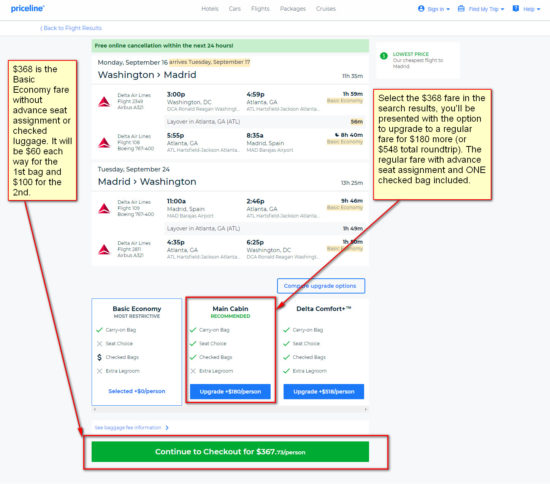Here is a highly detailed and cleaned-up caption for the given image:

---

**Screenshot of Priceline Flight Booking Page**

At the top left corner, the website header displays the Priceline logo. On the right, navigation options include "Sign In," "Find My Trip," and "Help." The page emphasizes a free online cancellation policy available within the next 24 hours.

**Flight Itinerary:**

- **Outbound Flight:** 
  - Departure: Monday, September 16
  - Arrival: Tuesday, September 17
  - Route: Washington, DC to Madrid, Spain
  - Listed Flights: 
    - **Delta Airlines:** 
      - Flight 1: 3:00 PM from Washington, DC to Atlanta, GA (1 hour 59 minutes)
      - Flight 2: 5:55 PM from Atlanta, GA to Madrid, Spain (8 hours 40 minutes)

- **Return Flight:** 
  - Departure: Tuesday, September 24
  - Route: Madrid, Spain to Washington, DC
  - Listed Flights:
    - **Delta Airlines:** 
      - Flight 1: 11:00 AM from Madrid, Spain to Atlanta, GA (3 hours 46 minutes)
      - Flight 2: 4:35 PM from Atlanta, GA to Washington, DC (1 hour plus an unspecified number of minutes)

**Highlighted Fare Options:**

- **Basic Economy:**
  - Carry-on Bag: No
  - Seat Choice: No
  - Checked Bags: Extra Cost
  - Extra Legroom: No

- **Main Cabin (Highlighted in Red):**
  - Carry-on Bag: Yes
  - Seat Choice: Yes
  - Checked Bags: Yes
  - Extra Legroom: No

- **Delta Comfort Plus:**
  - Carry-on Bag: Yes
  - Seat Choice: Yes
  - Checked Bags: Yes
  - Extra Legroom: Yes

A red arrow points to a highlighted square with a text overlay instructing to select the 368th fare in the search results. This fare offers an upgrade option for $180 more, totaling $548 for a round trip with advanced seat assignment and one checked bag included.

**Payment and Fare Information:**

- A green rectangle outlined in red at the bottom reads "Continue to checkout for $367.73 per person."

**Additional Information:**

- A text bubble at the top with a red arrow highlights: "$368 is the basic economy fare without advanced seat assignment or checked luggage. It will cost $60 each way for the first bag and $100 for the second."

---

This caption ensures that all the relevant details from the screenshot are clearly represented and structured for easy understanding.